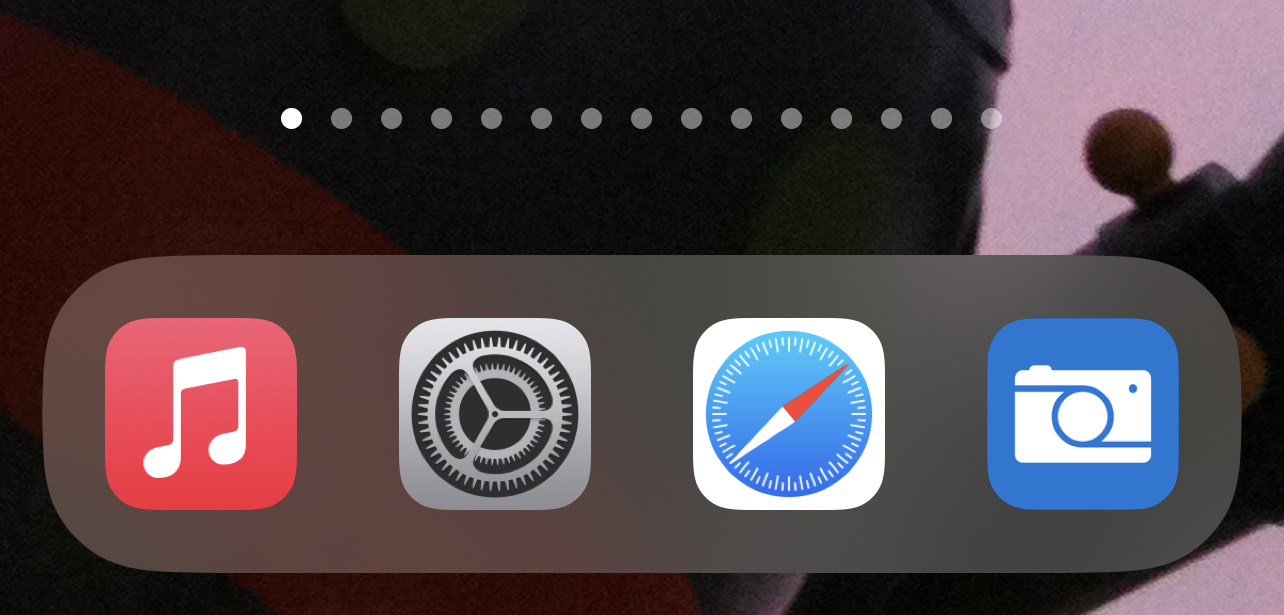This is an extreme close-up photograph of the lower portion of a smartphone screen. The left side of the screen features a dark background with an indistinguishable image, while the right side presents alternating bands of light purple and dark areas, followed by more light purple. Overlaying this background at the bottom of the screen is a semi-transparent, off-gray oval banner which houses four persistent app icons arranged from left to right. These icons include a music app, identifiable by its musical note symbol, the Settings app, Safari browser, and a Photos app denoted by a camera icon.

Above this oval banner is a series of indicator dots, suggesting the user has 15 different home screen pages, with the first one highlighted in white and the remaining 14 in gray. This visually implies that swiping horizontally will navigate through these various pages of applications. The close-up nature of this photograph emphasizes the detailed organization and layout of the user's smartphone home screen, particularly highlighting the user's choice of essential apps and navigation indicators.